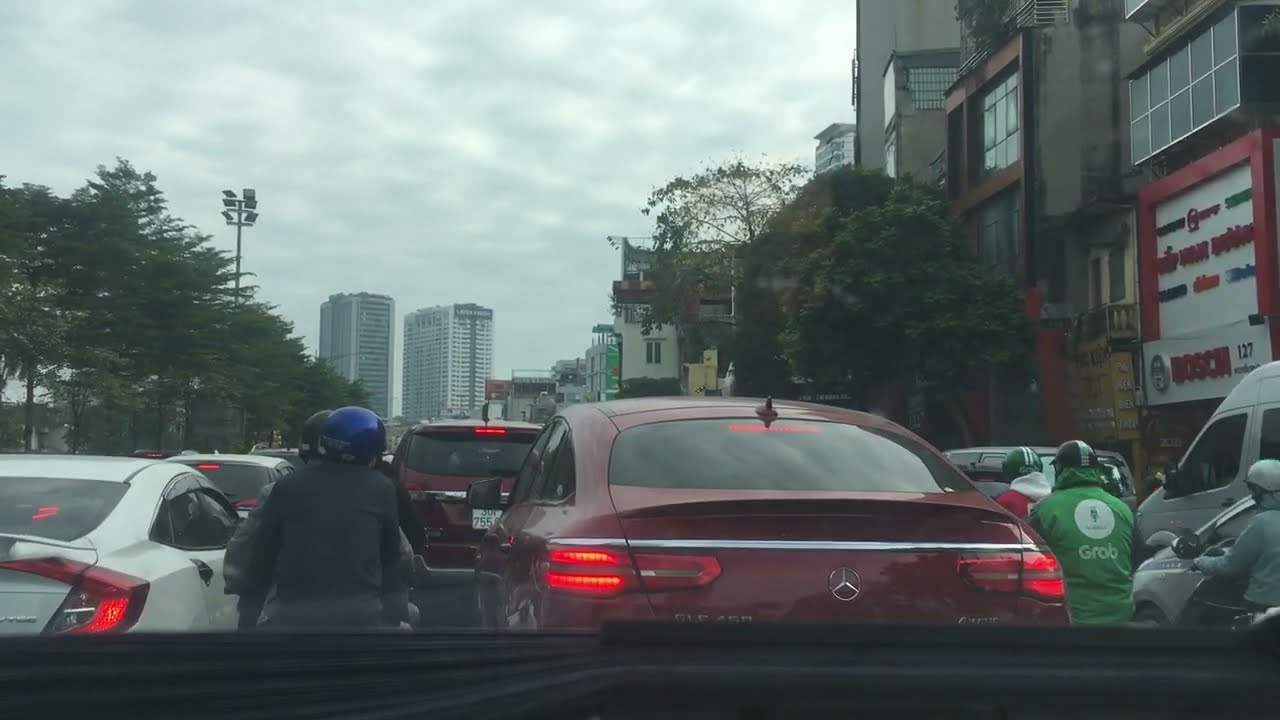The image, viewed from inside a vehicle through a slightly hazy windshield, reveals a busy street scene with a traffic jam. Dominating the middle of the picture is the back of a maroon Mercedes-Benz with its brake lights glowing. Immediately in front of it is another maroon SUV. To the left, the back end of a white sedan is visible next to a motor scooter with two helmeted passengers, one wearing a black helmet and black shirt, the other sporting a blue helmet. 

On the right side, beside the maroon car, there are at least two more motor scooters. One scooter rider is identifiable by a green helmet with white stripes and a red shirt, while another wears a green jacket with a black helmet featuring white stripes. A third rider in a gray sweater can be noticed further along, and a white van sits to the far right.

Tall buildings, possibly shops, line either side of the street, and in the distance, several taller buildings stand against a backdrop of a blue sky dotted with numerous small clouds. There are some trees visible on the sides, adding to the urban landscape's depth.